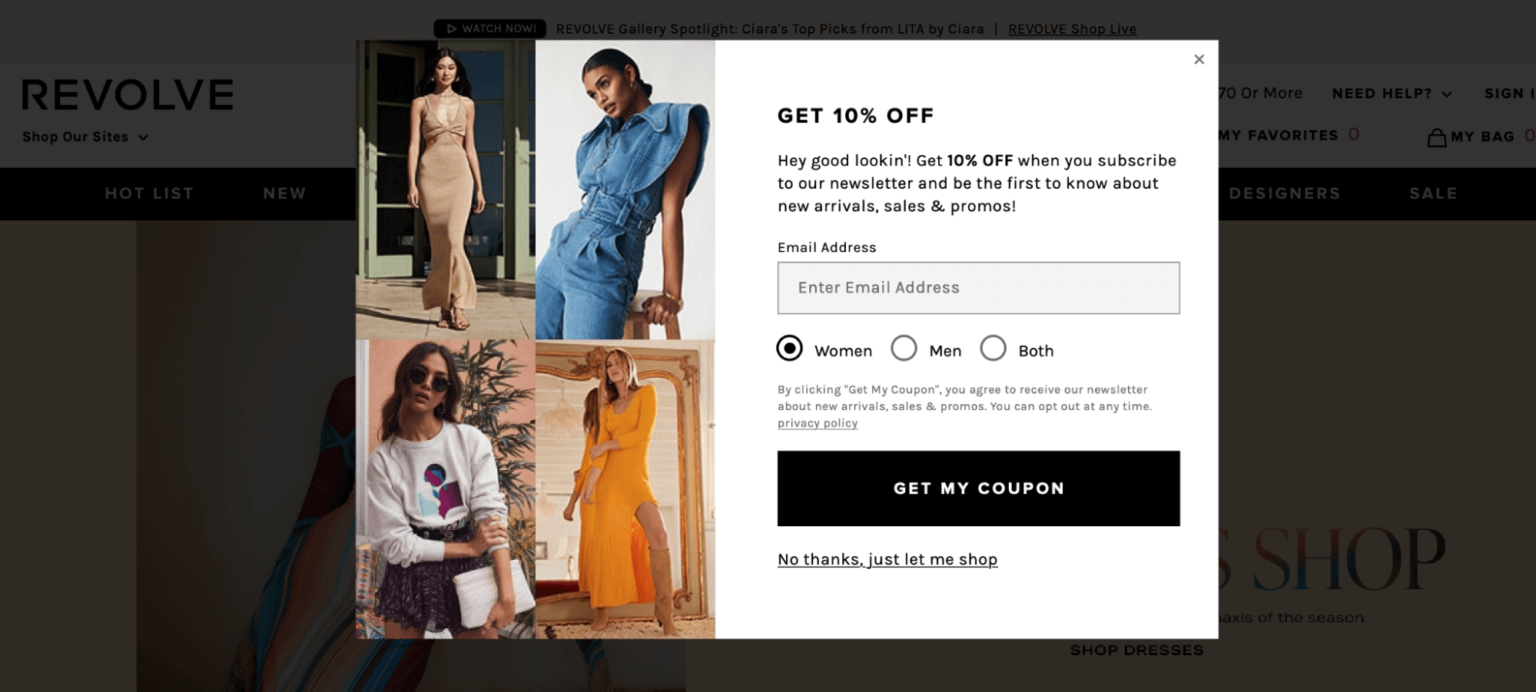The image appears to be a snapshot from the Revolve website, showcasing a promotional pop-up. At the top of the page, there are navigational links labeled "Hot List," "New," and more, accompanied by promotional headings such as "Revolve Gallery Spotlight" and "Clara's Top Picks from Lolita by Sierra." 

Dominating the foreground is a pop-up advertisement offering a 10% discount. The pop-up's design features a grid of four stylish models dressed in fashionable attire, arranged in a two-by-two layout. Positioned to the right of these images, the pop-up text reads: "Hey good looking, get 10% off when you subscribe to our newsletter and be the first to know about new arrivals, sales, and promos."

Beneath this message, there is a field to enter an email address and options to select interests in women's, men's, or both categories of fashion. The showcased viewer has selected the "women" option. A prominent black button labeled "Get My Coupon" is available to finalize the subscription.